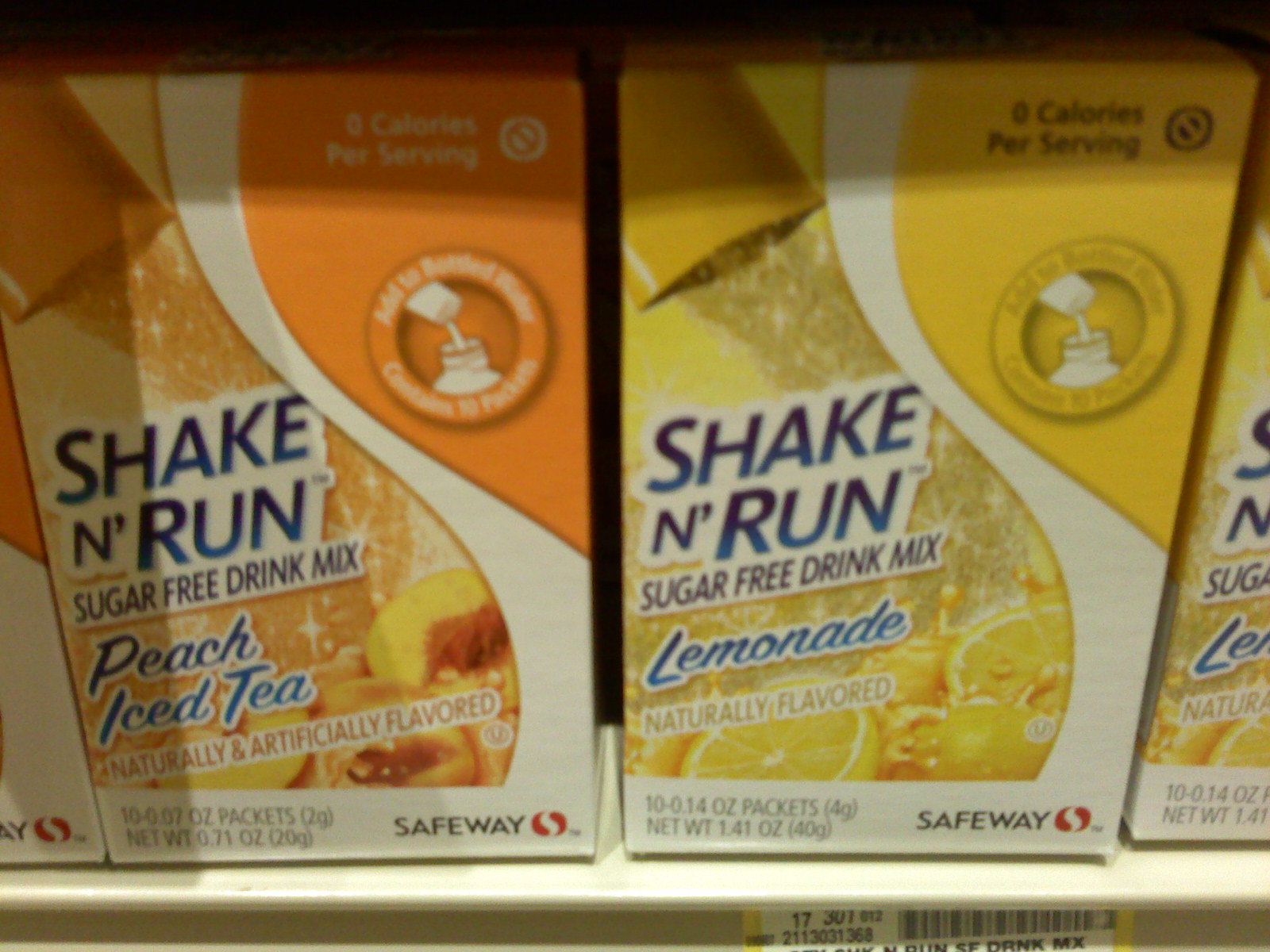This photograph captures a display in a Safeway store, showcasing their branded Shake and Run sugar-free drink mixes. The photo features two distinct drink mix packets prominently positioned on a store shelf. The first packet, designed with a striking combination of orange, navy, and white colors, is labeled "Peach Iced Tea." The second packet, bearing navy, white, and yellow hues, is labeled "Lemonade."

Both packets feature the word "Navy" on the front, accompanied by the product name, "Shake and Run sugar-free drink mix." At the bottom of each packet, the Safeway brand is marked in black, along with the recognizable red and white Safeway logo. Each of these drink mix packets contains 10 individual servings, with each serving weighing 0.14 ounces.

Below the neatly displayed drink mixes, a white metal shelf extends into the frame, providing a stable base for the products. Attached to this shelf is a black, yellow, and white price sticker, adding a dash of retail context to the image.